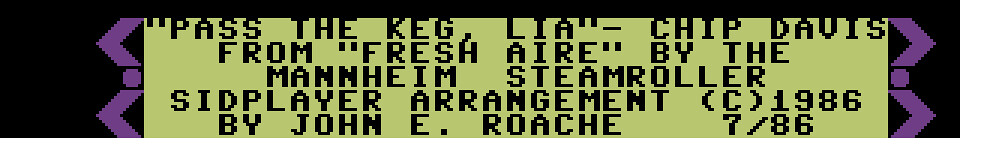The image captures a horizontal slice from a computer screen, set against a black or dark purple backdrop. The focal point is a large, yellow rectangle placed centrally within the frame. Black text within the rectangle reads: "That's the keg, Leah," followed by "Chip Davis" and "From 'Fresh Aire' by the Mannheim Steamroller," along with "Sid Player Arrangement" and "(C) 1986 by John E. Roache." There are distinct visual elements flanking the yellow rectangle: on both the left and right sides are columns featuring two light purple arrows pointing outward with a purple circle situated between them. This arrangement, with its contrasting colors and structured text, suggests a digital bulletin or some form of copyrighted material displayed on a computer screen.